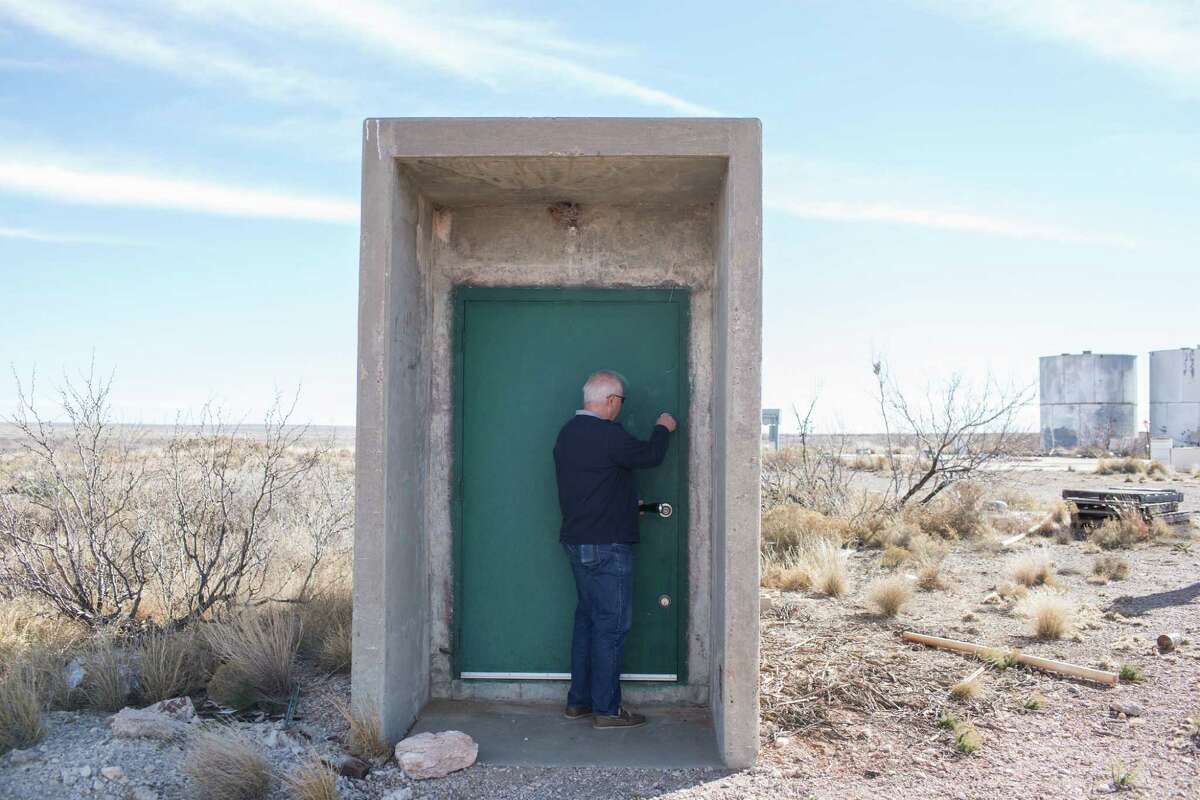In the middle of a scrubby desert landscape stands a peculiar gray concrete structure with an overhanging roof and walls, housing a prominently green door with a silver handle. The terrain surrounding the structure is a rough mix of dirt, sand, dead leaves, branches, and patches of tan grass, accentuating the stark contrast of human-made elements amidst nature. Off to the right, two rounded, gray metal tanks rise from the ground, possibly indicating an underground facility, with what looks like an air vent beside them.

An older gentleman is positioned directly at the green door, slightly balding with white hair, and wearing a long-sleeve navy shirt and loose-fitting blue jeans. His thin-rimmed glasses catch some light as he raises his right arm, appearing to knock or perhaps turn a key in the lock of the enigmatic door. The clear blue sky with a few long, thin clouds stretches above, encapsulating the surreal scenery in bright daylight. The photograph captures the man at the center, embodying a sense of curiosity and mystery as he interacts with the unexpected structure in this desolate field.